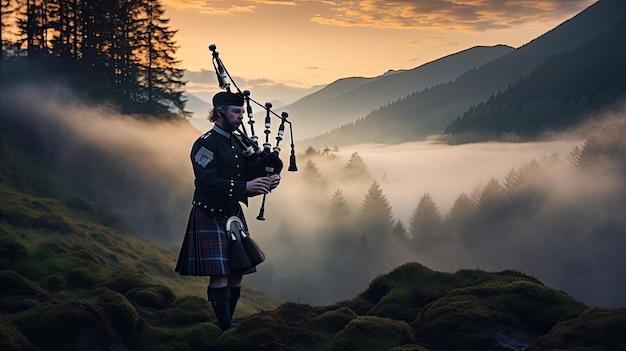This image captures a Scottish man playing the bagpipes, standing on a grassy, moss-covered hillside. The man is dressed in traditional Scottish attire, including a plaid kilt and a dark blue vested uniform adorned with several buttons and a blue crest on his right arm. He is also wearing black boots that reach almost to his knees and a hat strapped securely to his head. The scene around him is serene and atmospheric, with a foggy backdrop that includes a shimmering lake bordered by evergreen trees and towering mountains. The sky is partially obscured by clouds, and the lighting suggests either dawn or dusk, adding to the tranquil mood of the setting.